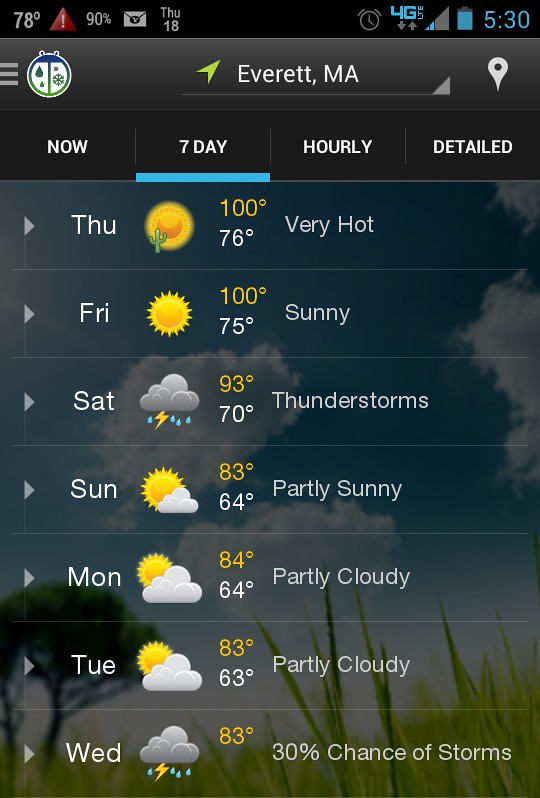This is a detailed weather forecast image for Everett, Maine, captured as a screenshot from a phone. The forecast spans seven days from Thursday to Wednesday, showcasing daily high and low temperatures, weather conditions, and additional mobile interface details. The backdrop features a background image of a sky with puffy clouds, green trees, and long grass.

Thursday and Friday both show a high of 100 degrees and a low of 76 and 75 respectively, with clear sunny icons indicating very hot weather. Saturday has a high of 93 degrees and a low of 70 degrees, with a cloud and lightning icon indicating thunderstorms. Sunday’s forecast is partly sunny with a high of 83 degrees and a low of 64 degrees, while Monday shows partly cloudy skies with temperatures around 84 and 64 degrees. Tuesday continues the partly cloudy trend with a high of 83 and a low of 63, and Wednesday, forecasted at 83 degrees, includes a 30% chance of storms indicated by a cloud with lightning and rain icon.

Additional details show that the screenshot was taken with limited cellular reception at 5:30, with the phone displaying indicators for 4G LTE connection and an ambient temperature of 78 degrees at the top left corner. The display is organized in columns under labels like “7 day hourly” and “detailed.”